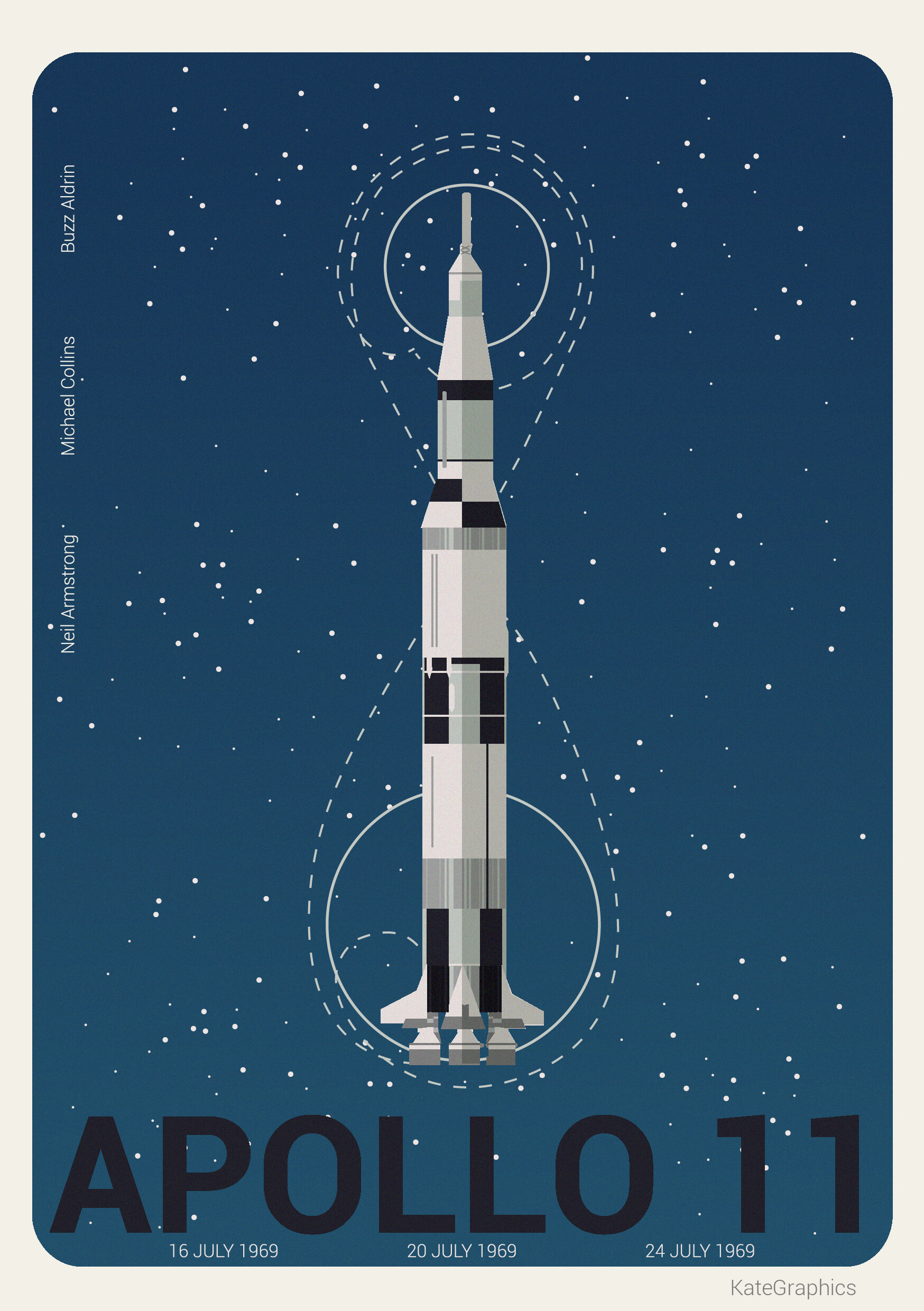The image is a detailed computer art illustration of the Apollo 11 rocket, presented in portrait mode. The central focus is on the rocket, depicted in shades of gray, black, silver, and white, pointing upwards. Surrounding the rocket is a diagram showing the Earth, Moon, and the path the spacecraft took during its historic mission. The background transitions from light blue at the top to dark blue at the bottom, with an array of white dots representing distant stars, giving it a night sky effect. Along the left side, the names of the astronauts, Neil Armstrong, Michael Collins, and Buzz Aldrin, are inscribed in small white font. Dominating the bottom is the title "Apollo 11" in large black letters, and beneath it are the dates of key mission events: July 16, 1969 (launch), July 20, 1969 (moon landing), and July 24, 1969 (Earth return), in smaller text. The overall composition resembles a commemorative card, capturing the essence of the Apollo 11 mission with a blend of illustrative detail and informative text.